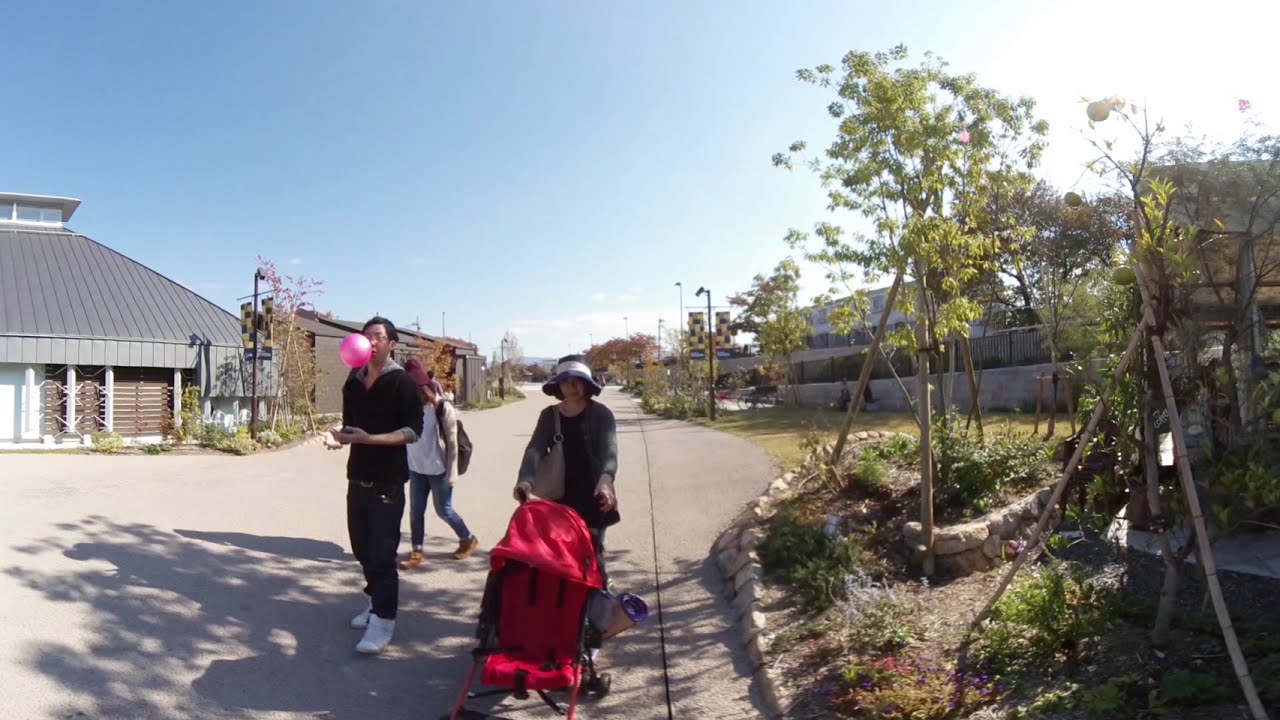The image captures an outdoor scene on a bright, clear day, featuring several people walking along a wide concrete pathway. In the center, a woman wearing a black and white bucket hat and a light gray jacket over black clothes is walking towards the camera. She has a purse draped over her left shoulder and is pushing an empty red stroller. To her left, a man dressed in a black hoodie, black pants, and white shoes is throwing a pink ball, which hovers at face level. Behind him stands another person, partially obscured, in a white long-sleeve shirt and blue jeans. The left side of the image showcases several buildings with metal siding and roofs, while the right side is lined with small, sparsely arranged trees and plants supported by artificial poles, some bearing green foliage and fruit. In the background, a building with a fence is slightly elevated on concrete. The clear blue sky overhead emphasizes the pleasant outdoor atmosphere.